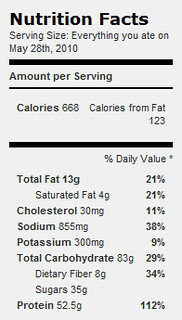The image depicts a black-and-white nutrition label set against a gray background. The label is titled "Nutrition Facts" and features the serving size as "everything you ate on May 28, 2010." Below the title, a black line separates sections, starting with "Amount per serving." It lists the following nutritional content: 668 calories, with 123 calories from fat. The total fat content is 13 grams, constituting 21% of the daily value, and includes 4 grams of saturated fat, also 21%. The cholesterol level is listed at 30 milligrams (11%), while sodium is noted at 855 milligrams (38%). Potassium is given as 300 milligrams (9%). The label further details total carbohydrates at 83 grams (29%), dietary fiber at 8 grams (34%), sugars at 35 grams, and protein at 52.5 grams, which amounts to 112% of the daily value. Quite humorously, it compresses an entire day's intake into one serving, offering a comprehensive snapshot of one's nutritional consumption on that specific date.